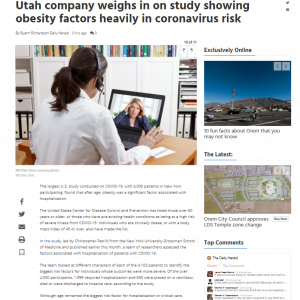Here is a cleaned-up and detailed descriptive caption for the image:

---

The image shows a busy online article interface with a predominantly white background. The layout is roughly square, slightly taller than it is wide, and features no borders. In the top-left corner, there is a headline in bold black font spanning two rows. The headline reads, "Utah company weighs in on studies showing obesity factors heavily in coronavirus risk," with only the "U" in "Utah" capitalized. This headline takes up about 80% of the top section, leaving an empty space to the right where two vertically stacked gray circles are visible.

Beneath the headline, on the left side, is a very small line of gray text, likely containing the author's name and the publication date, though it is too minuscule to be legible. Below this text is a large landscape-oriented photograph, approximately 20% wider than its height. The photograph captures the back of a woman with dark black hair in a ponytail, seated at a light brown wooden table. She wears a long-sleeved white shirt and headphones, and is looking at a laptop screen. On the laptop screen, another woman, possibly in a dark business suit with dirty blond or light brown hair, can be seen, with a backdrop of a bookshelf filled with books and videos.

The main article content below the photograph consists of five paragraphs in small gray text, each left-justified and varying in length from one to nearly four lines. On the left margin of this content, five vertical icons are aligned: Facebook, Twitter, an email envelope, and two unidentified icons.

The right third of the image features an additional panel. At the panel's top, the header "exclusively online" is displayed in left-justified bold font with a blue underline. Below this header is a landscape image of an outdoor scene with a blue sky and brown hilly terrain. Beneath the image are one and a half lines of illegible text.

Further down, another section titled "the [unreadable text]" (with the first word starting with an 'L') displays an overhead, full-color map, possibly of a park and its surrounding roads. Underneath the map is another snippet of small, unreadable text.

At the bottom of the panel, a header titled "top comments" appears, also in left-justified bold font with a blue underline. This section contains four or five user comments, each accompanied by an icon of a person and respective bold names, though the accompanying gray text is not readable.